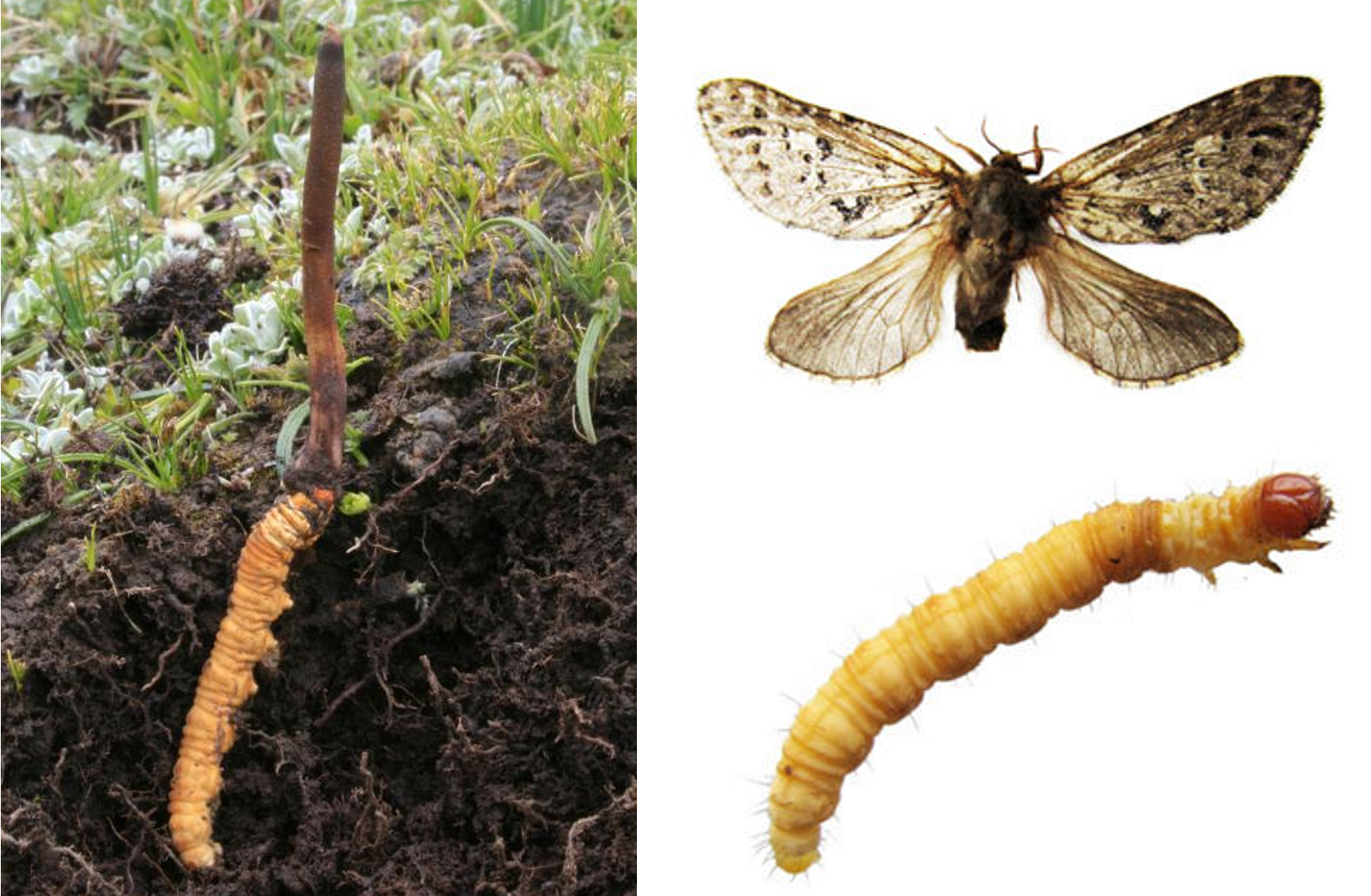The photograph is a composite of two images arranged side by side. Both images are in portrait orientation. The left image features a backdrop of dark brown dirt and mulch, with a goldish, creamish, orangey worm vertically positioned in the bottom half. The upper half showcases an array of grass, weeds, and rocks. The right image provides a closer view of the same worm, emphasizing its side profile, including its legs and fine hairs, revealing a red head. Above this worm, a moth with dark brown and black wings, and hints of white, can be seen. The overall clarity and brightness of the images suggest they were taken in well-lit conditions.